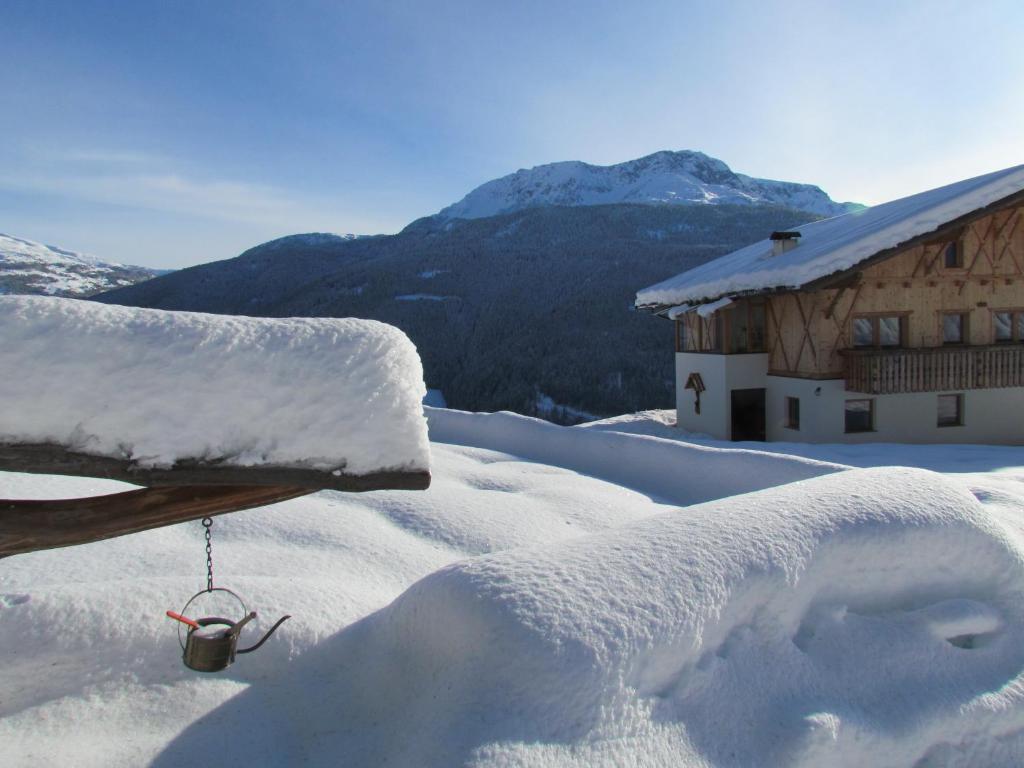The photograph captures a serene winter landscape in a mountainous region, likely mountainous Italy. The scene is cloaked in a thick, fluffy blanket of snow, extending from the foreground to the distant mountains. Towering in the background, the mountains are capped with pristine white snow beneath a striking blue sky streaked with clouds. 

Dominating the right side of the image, a charming cabin with a tan-colored, snow-laden slanted roof, brown structure, and cement foundation stands prominently. The cabin features at least two floors and a balcony, appearing relatively new. In contrast, the large, snowy landscape around it underscores the cabin's modest size. 

In the foreground, an intriguing wooden post or arm is heavily covered in snow, with a small silver trinket or oil can hanging from it, and an orange stick protruding from the pitcher. The post lacks a mailbox, featuring just the snowy end. The entire scene is devoid of people, amplifying the peaceful, untouched beauty of this winter wonderland.